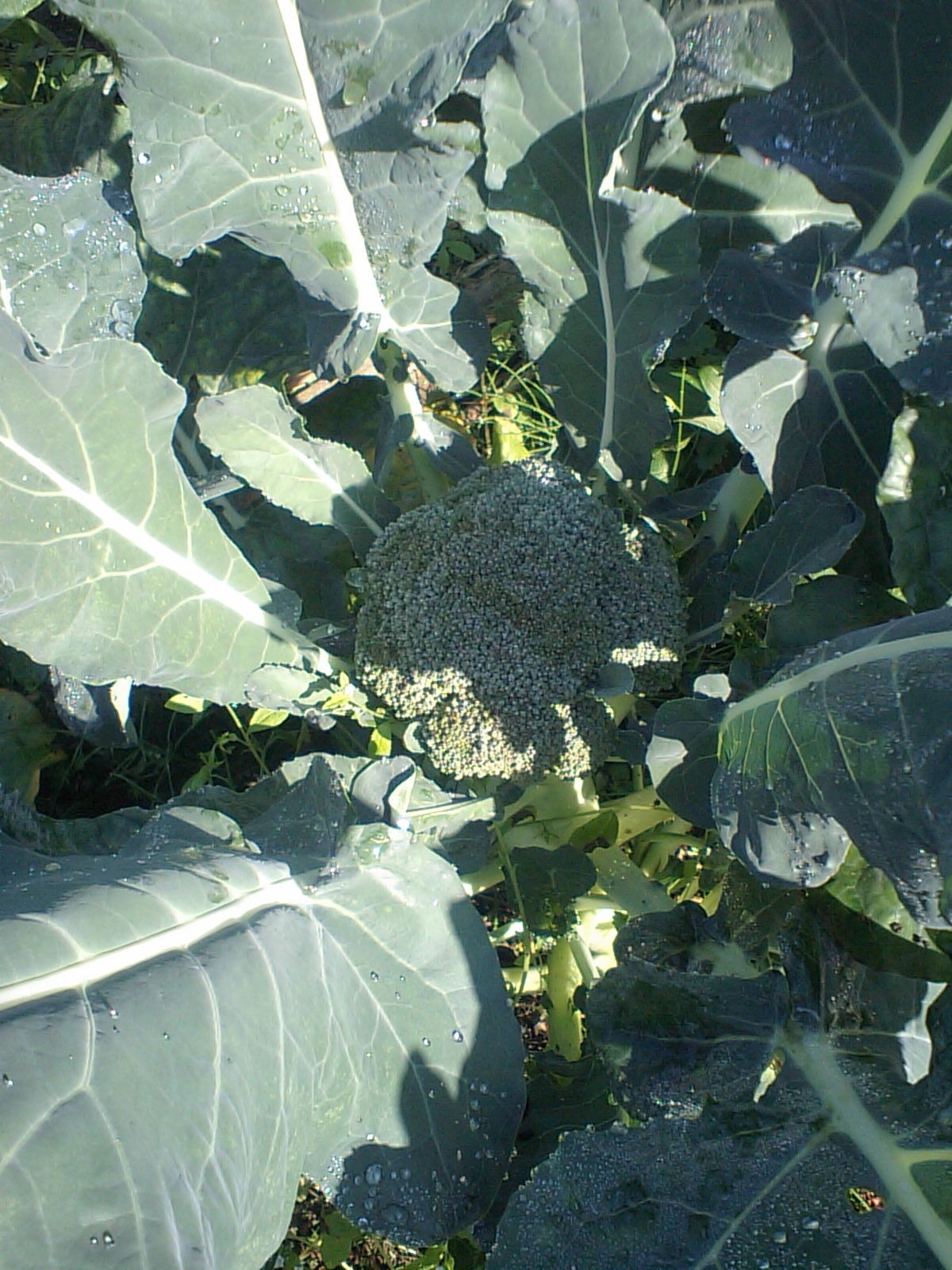This close-up, top-down photograph captures a lush, leafy plant growing outdoors, with a focus on what appears to be a central head of broccoli. The middle of the image showcases the broccoli, a textured, round, dark and light green floret that resembles a tree canopy. Surrounding the broccoli head are large, expansive leaves, each approximately two and a half feet long and a foot and a half across. These leaves are characterized by a muted green color, accentuated with thick white veins running along their length, and smaller veining in a whitish-yellow hue.

The scene is sprinkled with detailed droplets of water on the leaves, suggesting recent rain or watering. Some of the leaves display minute white specks and small tears, hinting at potential insect activity. The sunlight filters in from the left, casting a gentle glow and soft shadows that create a dynamic range of light and shadow across the foliage. The plant is rooted in the ground, with visible soil, grass, and clovers beneath the broad leaves, indicating a healthy outdoor garden setting. The meticulous details, such as the dew and the interplay of sunlight and shadow, suggest the photo was taken in the early morning or mid-afternoon, capturing the serenity and freshness of the plant in its natural habitat.